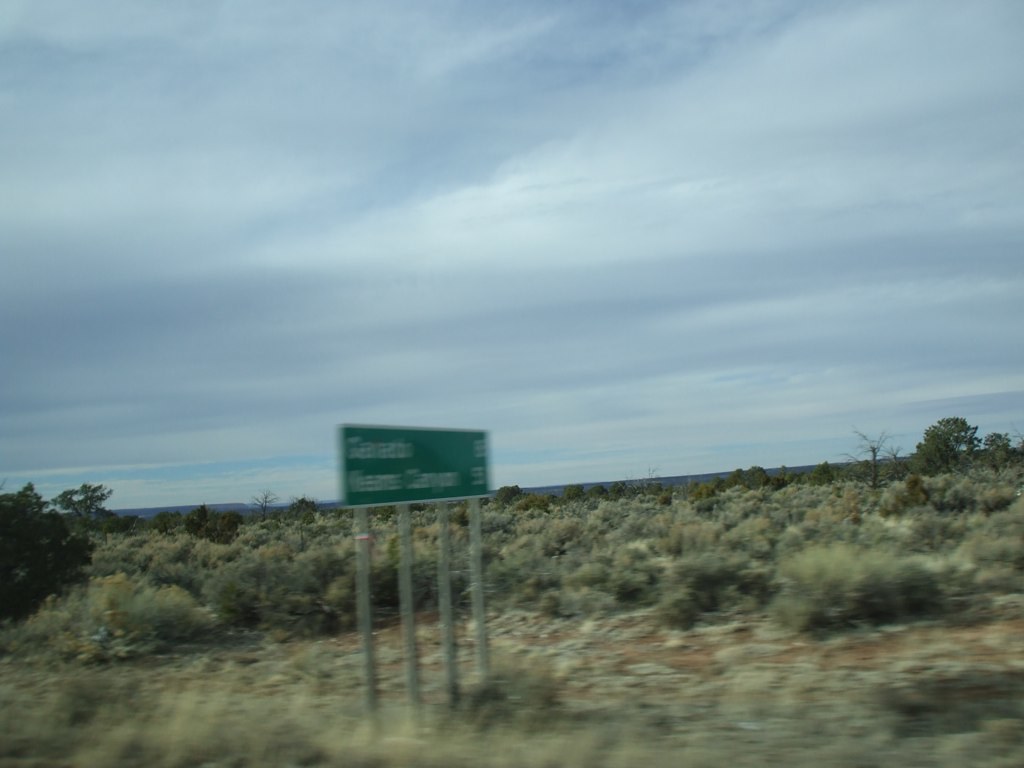A blurry photograph likely taken from a moving vehicle captures a desert scene dominated by a cloudy sky with wispy white clouds and patches of blue peeking through. The central feature is a green rectangular highway sign with white text that lists the names of two cities and the miles to each, though the writing is indistinguishable due to the blur. The sign is atypically supported by four vertical posts and is set amidst an arrid landscape characterized by dry, grayish-brown scrub vegetation and patches of cleared dirt. Larger, dark green trees and a leafless tree are visible in the background. Further back, an elevated structure possibly indicating a railroad right-of-way adds depth to the scene. The whole image suggests a moment in the Southwestern United States, reminiscent of landscapes along historic routes like Route 66.